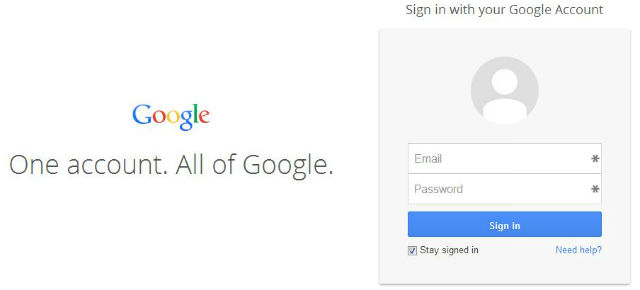This image depicts a Google sign-in screen from a web interface. The word "Google" is prominently displayed on the left side of the screen in its characteristic multi-color scheme: blue, red, yellow, and green. Directly below this, in a blackish-gray font, the phrase "One account. All of Google." is visible.

To the right of this, at the top, the text "Sign in with your Google Account" appears, also in blackish-gray. Beneath this header is a central light gray square. At the top center of the square, there is a circular avatar placeholder, which features a simplistic white icon representing a person, consisting of a white circle head and a basic body shape.

Below the avatar, there are two white text input fields stacked vertically. The first field is labeled "Email," and the second one is labeled "Password." Each field has a small asterisk on its right side, possibly indicating required fields. 

Further down, there is a wide, blue horizontal button with the text "Sign in" written in white. Adjacent to this button, to the left, is a small checkbox labeled "Stay signed in." To the right of the checkbox, the words "Need help?" are written in blue, followed by a question mark.

Overall, this image captures the login interface for accessing a Google account.